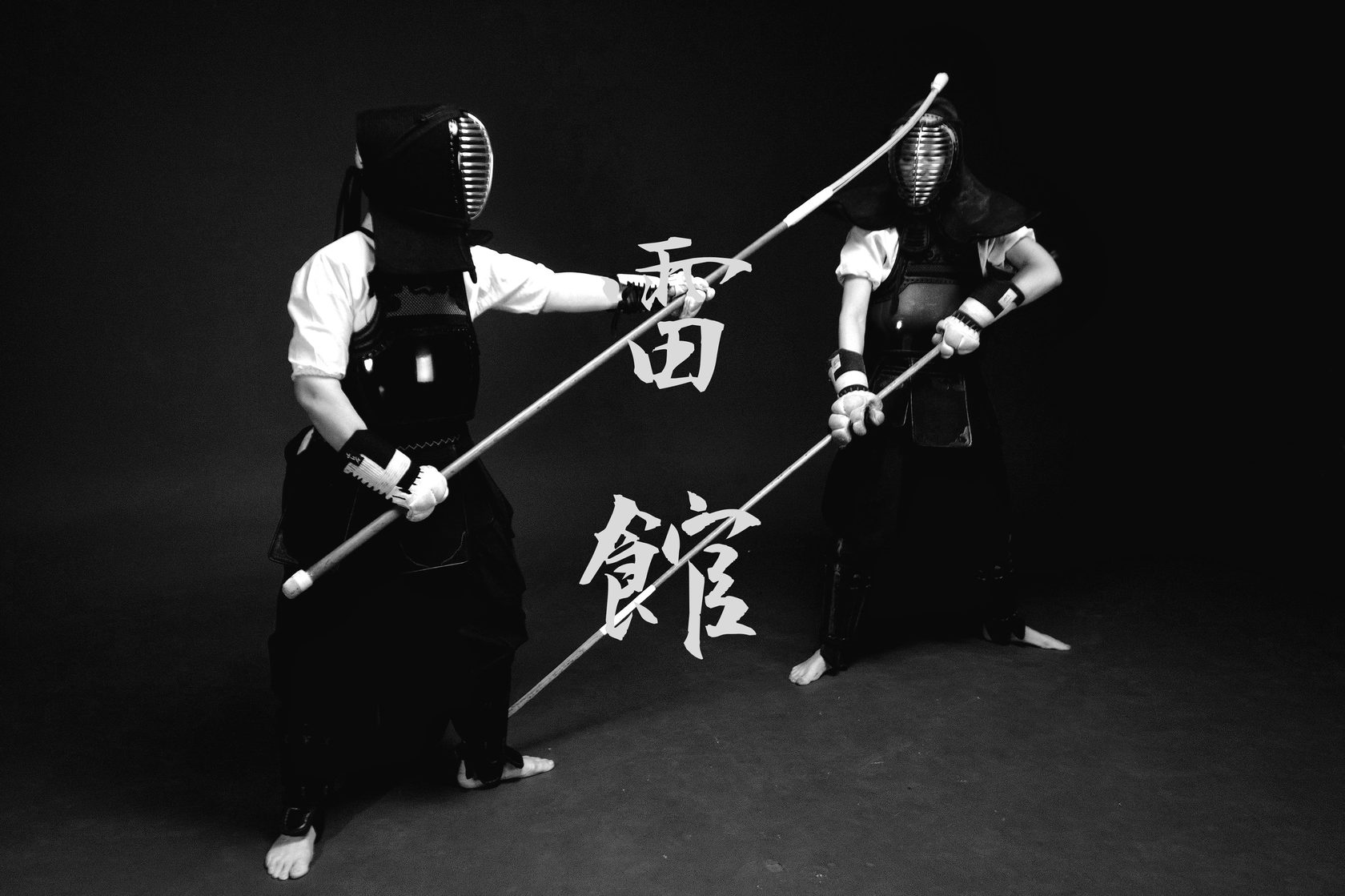This black-and-white photograph features two individuals clad in traditional martial arts gear, engaged in what appears to be a demonstration. Both are wearing distinctive black garments resembling a hybrid of overalls and aprons, silhouetting against a dark background. Underneath these outfits, they sport short-sleeved white shirts or shirts with sleeves rolled up, along with long padded gloves. Their heads are protected by hooded masks; the hoods are black while the masks feature a metallic or silver grill that obscures their faces entirely. 

Each of them is wielding a long, white baton-like weapon, which is straight but curves slightly at the ends, and they adopt martial arts stances indicative of combat—one appears to be poised to strike at an opponent's head, while the other seems ready to sweep a leg. Their positioning exudes a sense of fluid motion, capturing a moment of intense focus and skill. Despite their historical and cultural setting, their attire does seem to have some modern safety adaptations. Emphasizing their cultural roots, East Asian characters, specifically Chinese or Japanese, are seen at the center of the frame as well as on the weapons, grounding the image in its cultural context. The floor they stand on is cement, enhancing the contrast with their traditional yet modernized outfits.